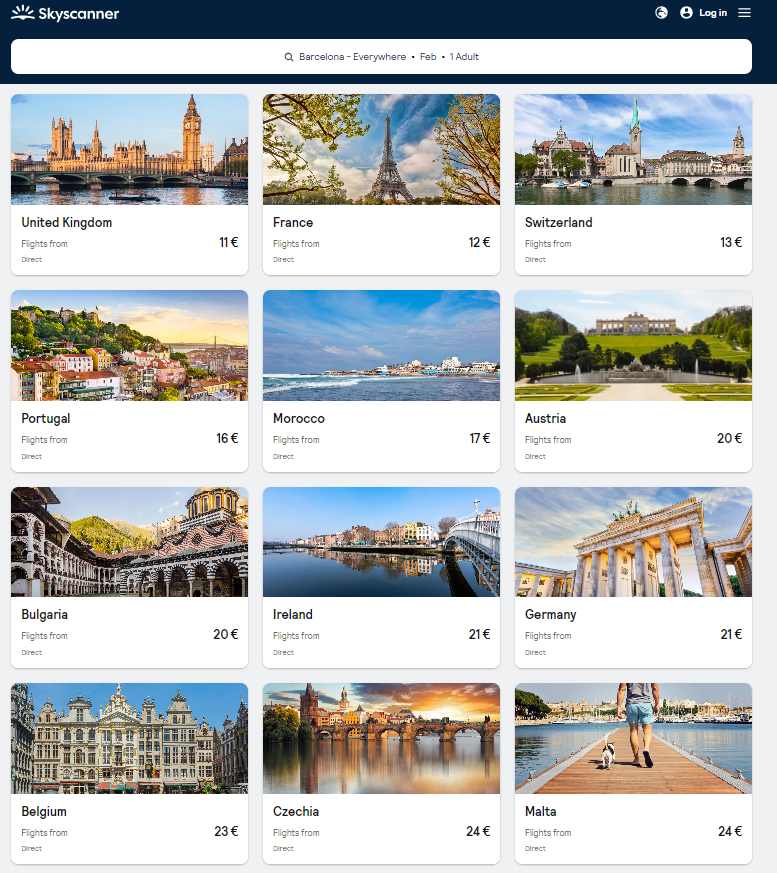The image is a screenshot of a computer graphic displaying a travel search interface. At the very top, there is a black border, and in the upper left-hand corner, the text "Sky Scanner" is visible. On the right side of this black border, there is a "Login" option.

Beneath the black border is a search bar in which someone has entered "Barcelona everywhere February 1 adult". Below the search bar, the interface displays several images organized into four rows, each containing three pictures.

In the first row:
1. The first image is labeled "United Kingdom" and has a price tag of 11 pence.
2. The second image features the Eiffel Tower and is labeled "France" with a price of 12 pence.
3. The third image shows a building exterior and is labeled "Switzerland" with a price of 13 pence.

In the second row:
1. The first image depicts a town on a hill and is labeled "Portugal" with a price of 16 pence.
2. The second image shows a city along the water labeled "Morocco" with a price of 17 pence.
3. The third image features a building with green grass in front of it labeled "Austria" with a price of 20 pence.

In the third row:
1. The first image shows a building with a mountain in the background and is labeled "Bulgaria" with a price of 20 pence.
2. The second image depicts a city alongside a body of water labeled "Ireland" with a price of 21 pence.
3. The third image features a building with large columns and is labeled "Germany" with a price of 21 pence.

In the final row:
1. The first image shows a large building with a blue sky behind it, labeled "Belgium" with a price of 23 pence.
2. The second image depicts a water area with a bridge over it, labeled "Chechnya" with a price of 24 pence.
3. The final image features a boardwalk extending into the water and is labeled "Malta" with a price of 24 pence.